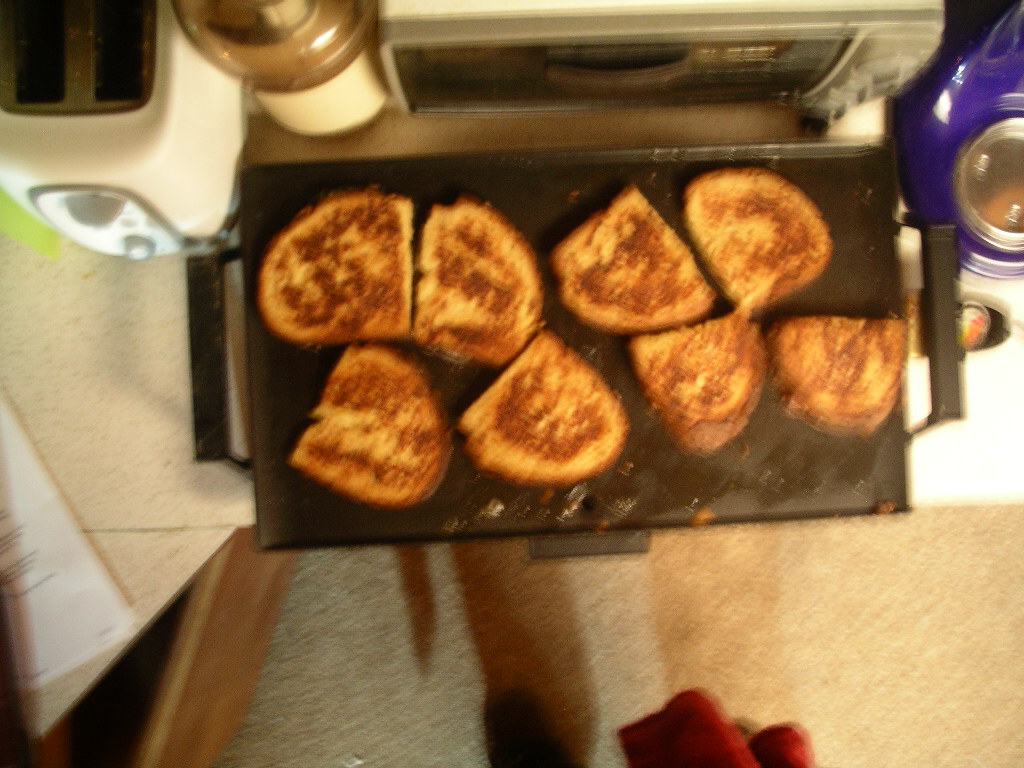This is a low-quality, blurry image taken from above, directly looking down into a kitchen scene. The main focus of the image is a rectangular brown baking sheet with eight pieces of oval-shaped, toasted French bread, each slice cut in half. The sheet is placed on a white countertop, which also holds various kitchen items. To the upper left corner, there is a white toaster, and beside it are a brown container, a gray microwave or toaster oven, and a purple container. The countertop has a piece of paper with indistinguishable writing on it. On the floor, which appears to be light-colored carpet, the shadow of the person taking the photo is visible, showing the bottom of their red pants or skirt and the tip of a black shoe.